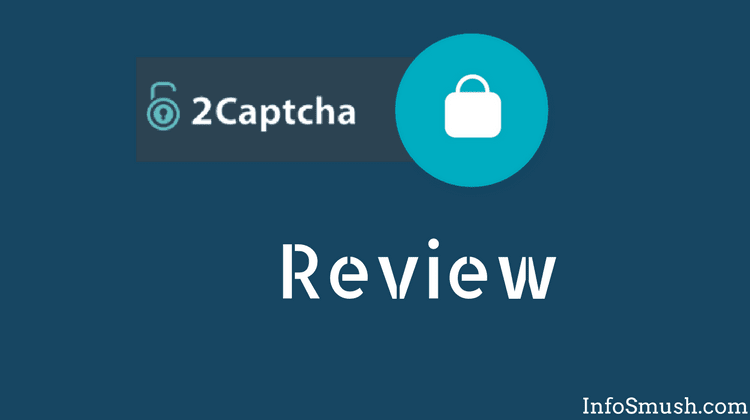This image is a screenshot, likely from a website. The background is a deep navy blue. Slightly off-center to the right, there is a prominent turquoise circle housing a small app icon that resembles a briefcase, characterized by its rectangular shape, curved edges, and rounded handle. To the immediate right of this circle, there is a black rectangle that features a blue padlock icon. Below this, a design element incorporates a series of turquoise circles, open at the top.

In bold white text, the phrase "To CAPTCHA" is displayed, followed closely below by the word "REVIEW" in larger letters. The letters in "REVIEW" have a unique design, featuring vertical cuts down the middle of several letters such as the R, top of the E, V, and so forth.

In the bottom right-hand corner of the image, the text "InfoSmush.com" is printed in white, identifying the source or creator of the content. The purpose of the phrase "To CAPTCHA Review" remains unclear without additional context, although it appears to be related to verifying or reviewing a CAPTCHA process.